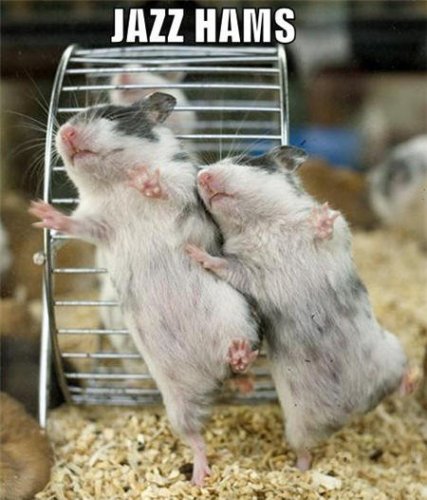This horizontally aligned photograph, potentially meant to be comical or a meme, displays a detailed scene of three hamsters in a cage. The cage features a silver metal hamster wheel in the background, inside which a blurry hamster can be seen. The wheel, cylindrical in shape, has about 20 thin metal bars or wires running horizontally across its top. The background of the image is somewhat blurred, with various objects: a white object at the top upper right, a blue object beneath that, and sections of black and white towards the right side. There's also a tan, soft disc shape at the bottom left and a brown shape in the upper left, possibly another hamster.

In front of the wheel, prominently displayed, are two hamsters appearing to execute a playful "dance" move reminiscent of jazz hands, with one leg raised and arms outstretched. The leftmost hamster has a white belly, pink feet, a pink nose, and clear white whiskers, with a black ear and eye visible. The second hamster, slightly smaller, has similar coloring but features more grey and black spots on the lower right belly.

The photograph is overlaid with white text bordered in black at the top, humorously captioned "Jazz Hams," playing on the phrase "jazz hands" and highlighting the hamsters' positioning. The image has a grainy quality, suggesting it might be older, possibly from the 70s or 80s, and could hail from the United States. The overall charm and playful nature of the image contribute to its potential status as a widely enjoyed meme.